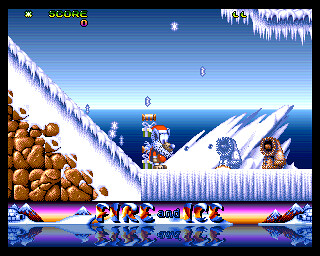This still from a video game showcases a wintry scene set on an iceberg. The lower quadrant of the screen features text, while the center prominently displays the words "fire" and "ice," both normally and as upside-down reflections in an icy body of water. The landscape is adorned with graphic representations of icicles and snow, evoking a chilly, frozen atmosphere. The predominant colors in this captivating scene include shades of blue, white, pink, purple, black, and brown, enhancing the wintry theme and creating a visually striking contrast.